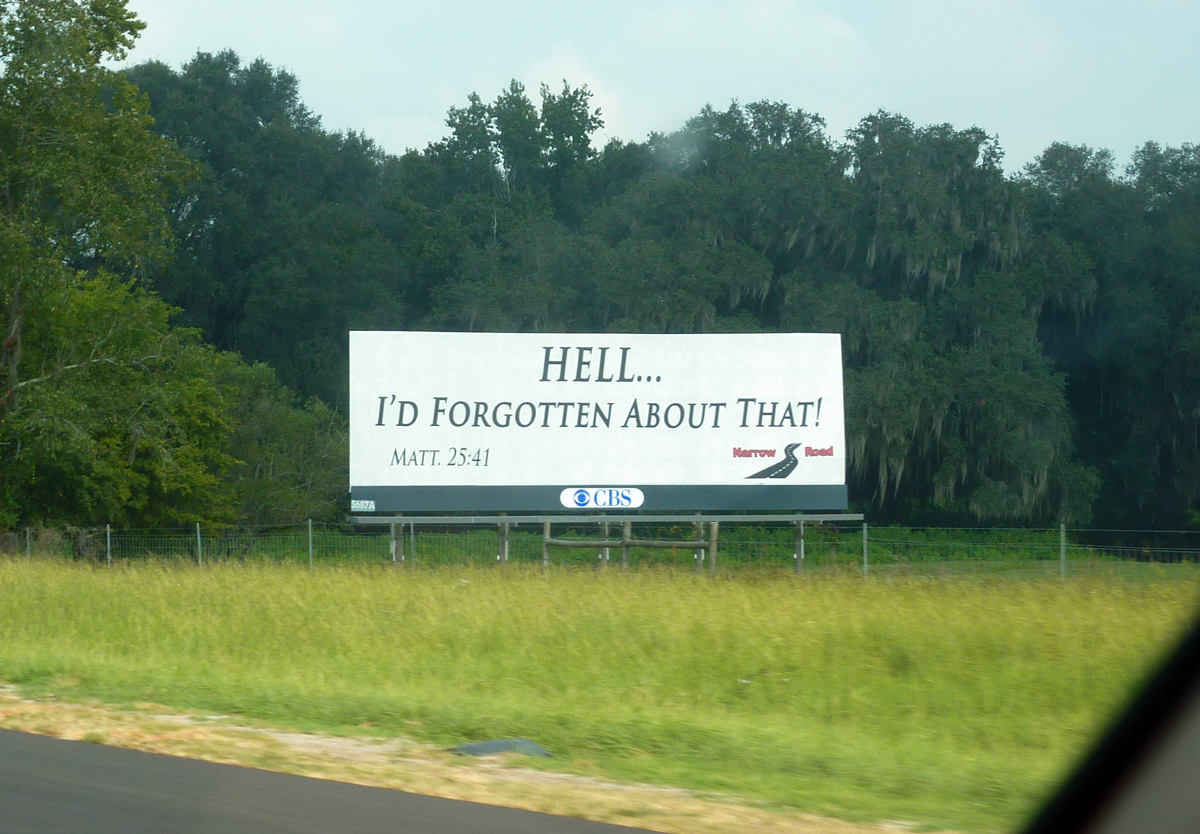This image captures a roadside billboard as viewed from inside a car, with part of the car frame and window visible along the bottom right edge of the photo. The billboard features a stark white background with a curious message in green lettering that reads, "Hell... I'd forgotten about that." Below this, on the left side, is a Bible reference: "Matt 25:41," suggesting a religious context, although the verse seems to be presented out of its broader scriptural narrative. The lower right corner of the billboard showcases a painted road that curves, flanked by the words "Narrow Road" in bold red letters. The billboard stands in a lush field of green grass, positioned alongside a highway. This apparent attempt at religious messaging invites travelers to ponder its meaning as they drive past.